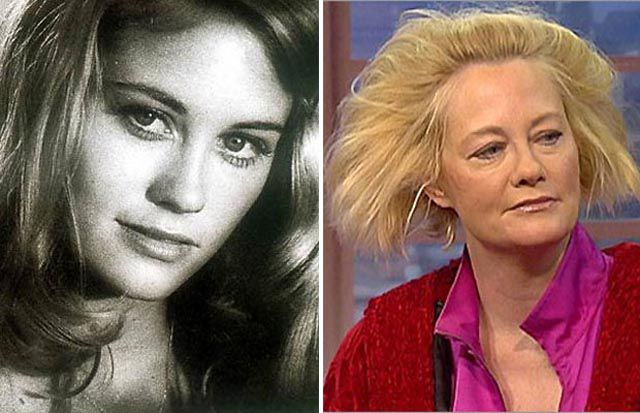This image consists of two juxtaposed photographs, each occupying an equal half of the frame, delineated by a solid white line down the center. The photograph on the left is an older black-and-white image from the 1960s of a young, blonde Caucasian woman with pale-colored eyes. Her face and hair dominate the frame, extending from her upper neck to her forehead. She possesses a seductive yet slightly innocent expression, characterized by a slight smile and minimal makeup, such as light mascara. Her hair is shoulder-length, loosely wavy, and voluminous, possibly adorned with a faint necklace barely visible or just her hair.

The photograph on the right appears decades later, likely from the 80s or early 90s, depicting an older Caucasian woman who might be the same person. She wears a red coat over a pink blouse, with both garments appearing soft and silky, respectively. Her hairstyle is a chin-length, stiff-looking bob, dyed blonde and seemingly styled with hairspray. Her makeup is understated, featuring light eyeliner and possibly some lip gloss. She looks pensively off to the viewer's right, her body angled slightly left, with a backdrop comprising a white windowpane opening onto an urban landscape. The window structure in the backdrop includes around six square panes and exhibits reflections of light, adding a modern, slightly talk-show atmosphere to the scene.